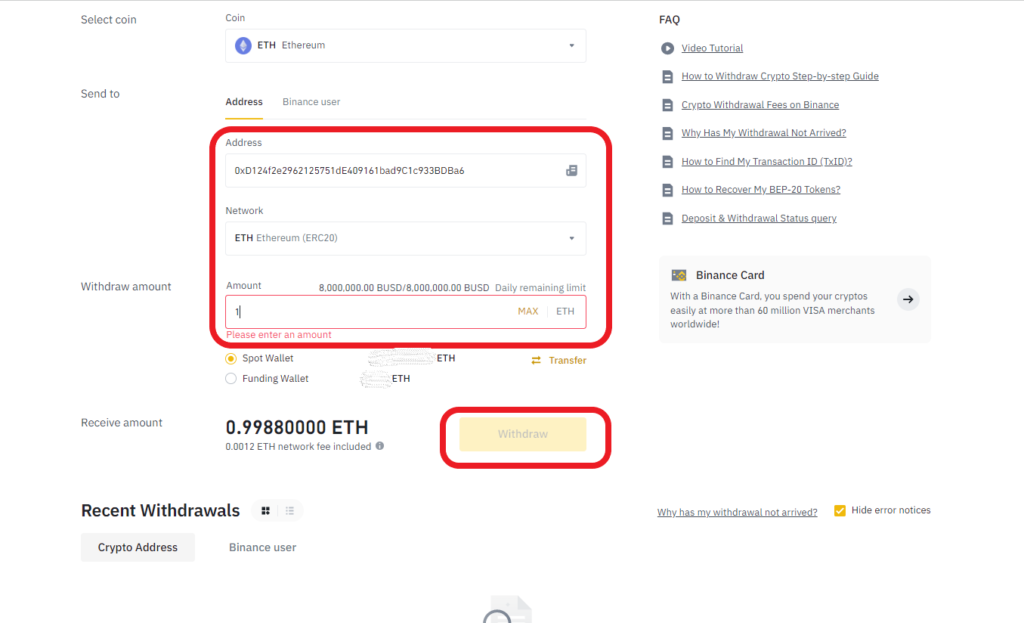The image features a user interface on a white background predominantly used for cryptocurrency transactions. Centered within a blue circle, the top section displays options: "SELECT COIN," which lists "COIN" and "ETH" (Ethereum). Below, the fields "SEND TO" and "ADDRESS" are highlighted, with the address area underlined in orange and enclosed in a red rectangle containing a series of letters and numbers.

Further down, the interface shows "NETWORK" with options "ETH" and "ETHERIUM," specifying "ERC20" in parentheses, indicating the Ethereum blockchain standard. The "AMOUNT" field is opened with a cursor visibly entering a value of "1." Adjacent to this, "MAX" is displayed in orange next to "ETH."

Beneath the amount input, a message reads "PLEASE ENTER an amount." To the left, "WITHDRAW AMOUNT" is titled above two selectable options: "SPOT WALLET" and "FUNDING WALLET." The "SPOT WALLET" button is filled in orange, indicating it's currently selected, with an associated balance amount that's scratched out and labeled in ETH.

At the bottom, there are directional indicators: an orange "TRANSFER" button with an arrow pointing to the right, and another arrow pointing to the left just below it. The image seems to guide users through the process of entering withdrawal or transfer details for a cryptocurrency transaction.